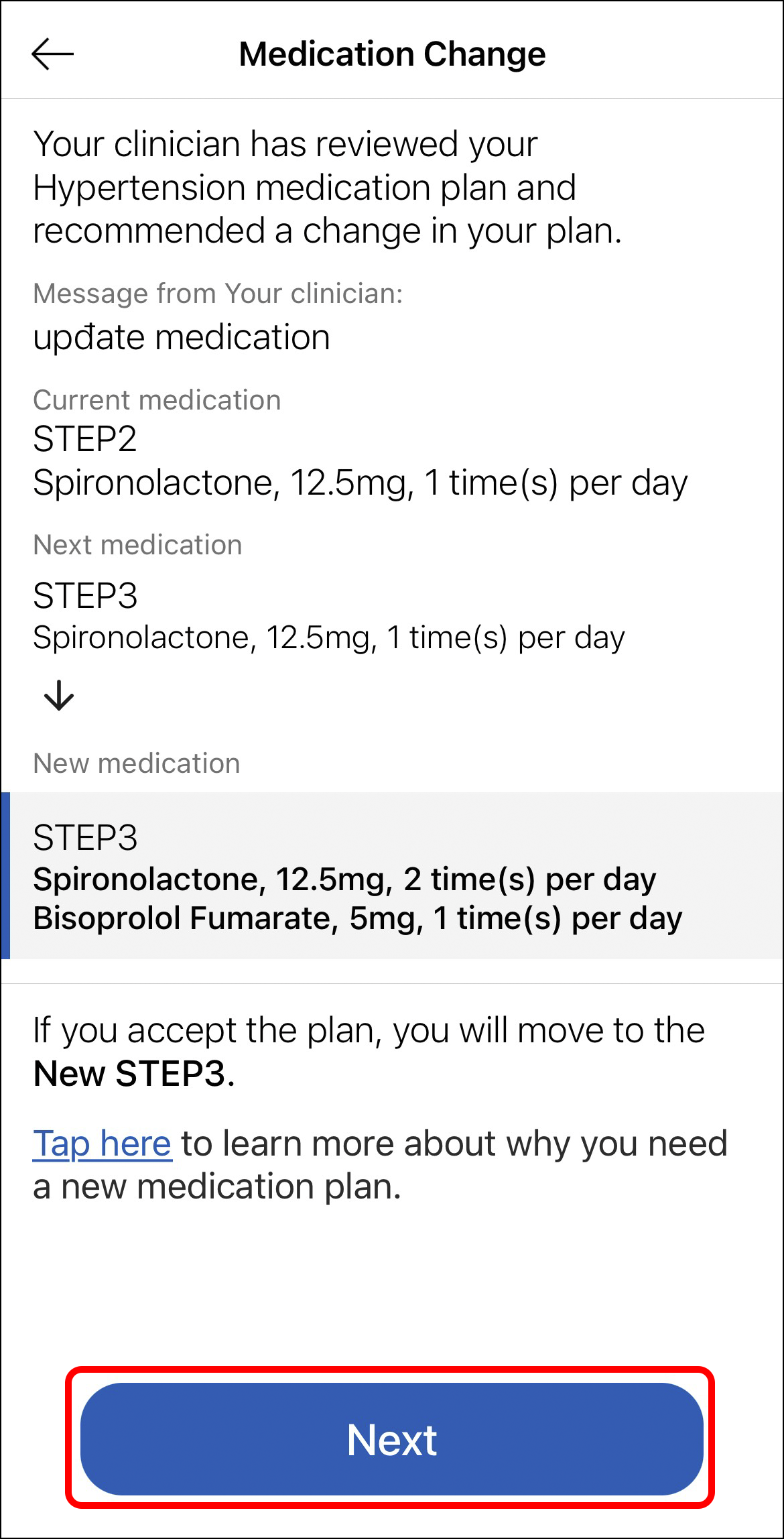Screenshot from a mobile app detailing a medication adjustment for a patient with hypertension. The screen displays a message stating that the patient's clinician has reviewed their hypertension medication plan and has recommended changes. The message from the clinician instructs an update to the current medication regimen: 

1. The current medication, "Spiroclit" (exact spelling unclear), initially prescribed once per day, will be increased to twice per day.
2. An additional medication will be added to the plan.

The interface suggests a step-by-step plan for the adjustments, indicating that if the patient agrees to the changes, they should tap the "Next" button, which is prominently circled in red.